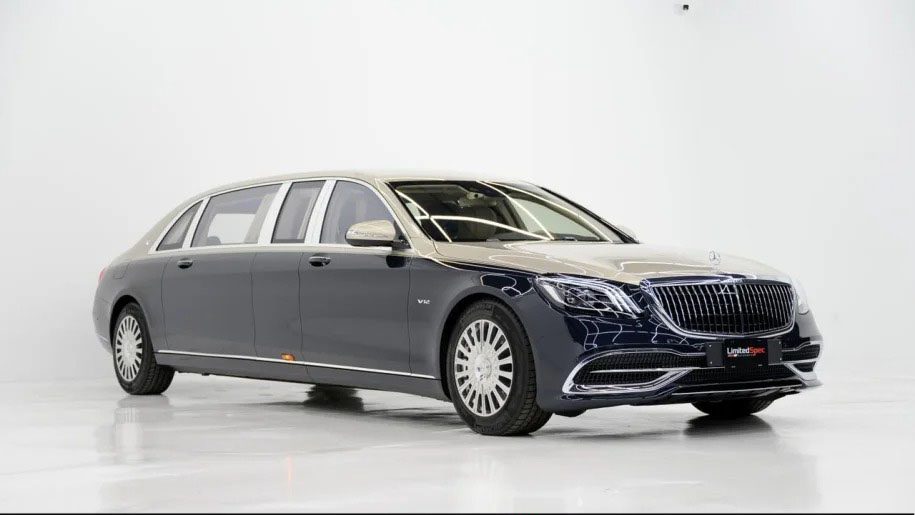A striking black and white photograph displays a high-end limousine, resembling a Rolls-Royce or Mercedes-Benz, diagonally parked on a glossy, white showroom floor. The car's sleek, extended black body contrasts with the reflective white surface, creating dramatic shadowing and reflections. An ornate yet inornate silver grille dominates the front, accompanied by a front license plate reading "limited spec" in white and red lettering on a black background. The hood and roof feature a distinctive lightning bolt design, adding to the car's luxurious aesthetic. Four uniquely-shaped windows span the cabin at the top, contributing to the sleek appearance, while partially raised windshield wipers rest on the gleaming front glass. Silver hubcaps with a spoke design reminiscent of wagon wheels adorn the black tires, enhancing the vehicle's sophisticated detail. There are no occupants visible inside the car, and the entire scene is set against a plain white wall, amplifying the grandeur of the vehicle.